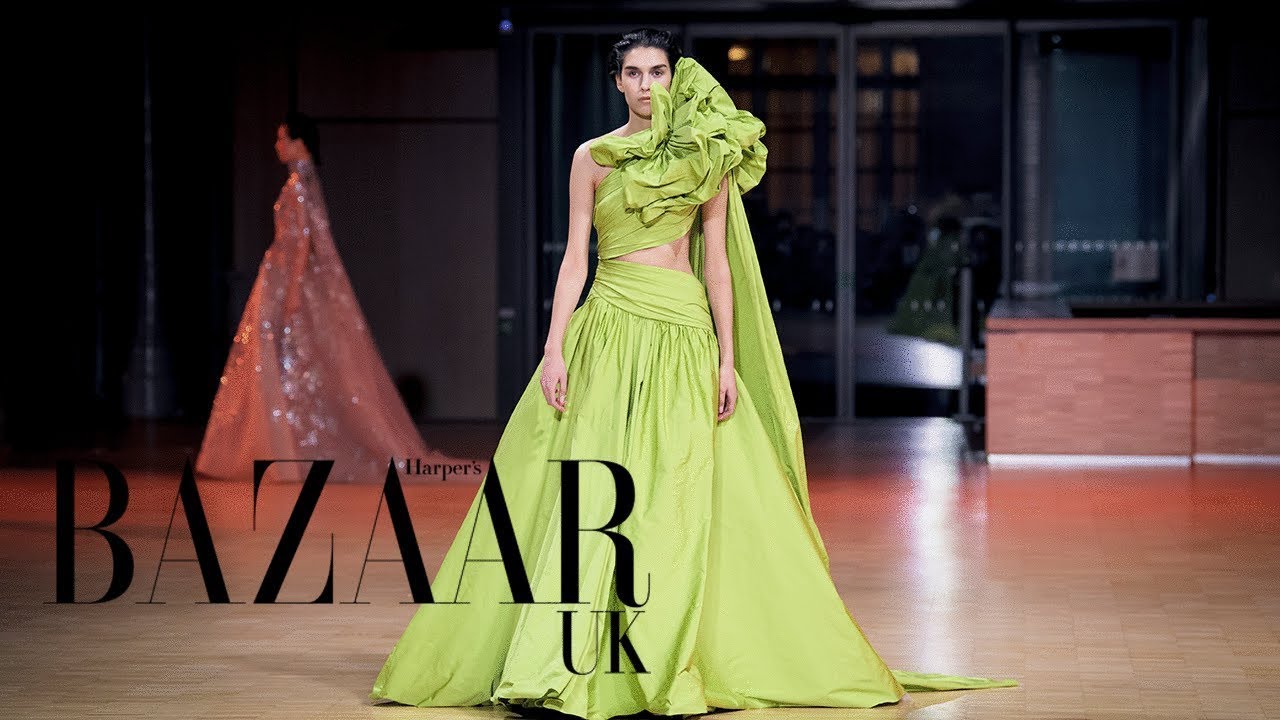In this horizontal rectangular color photograph, a model commands the runway, front and center, in an eye-catching lime green ball gown. The gown features a top that wraps around her body like a toga, creating a cutout at the waist before flowing into a voluminous ball gown. Adding to the dramatic flair, her left shoulder is adorned with an enormous ruffled bow, towering at four times the size of her head and extending into a train. The model, with her dark hair pulled back and arms bare, projects a neutral expression as she walks on a light-colored wooden floor. 

Behind her, slightly to the left, is another woman, possibly the previous runway model, dressed in a long, sparkly white gown with dark hair cascading down. The background is minimally decorated, with what appears to be floor-to-ceiling windows and perhaps a desk.

Dominating the image in bold, black capital letters is the text "Bazaar," with "Harper's" neatly placed between the two A's in "Bazaar," and "UK" underneath, suggesting that this photograph might serve as an advertisement for Harper's Bazaar UK.